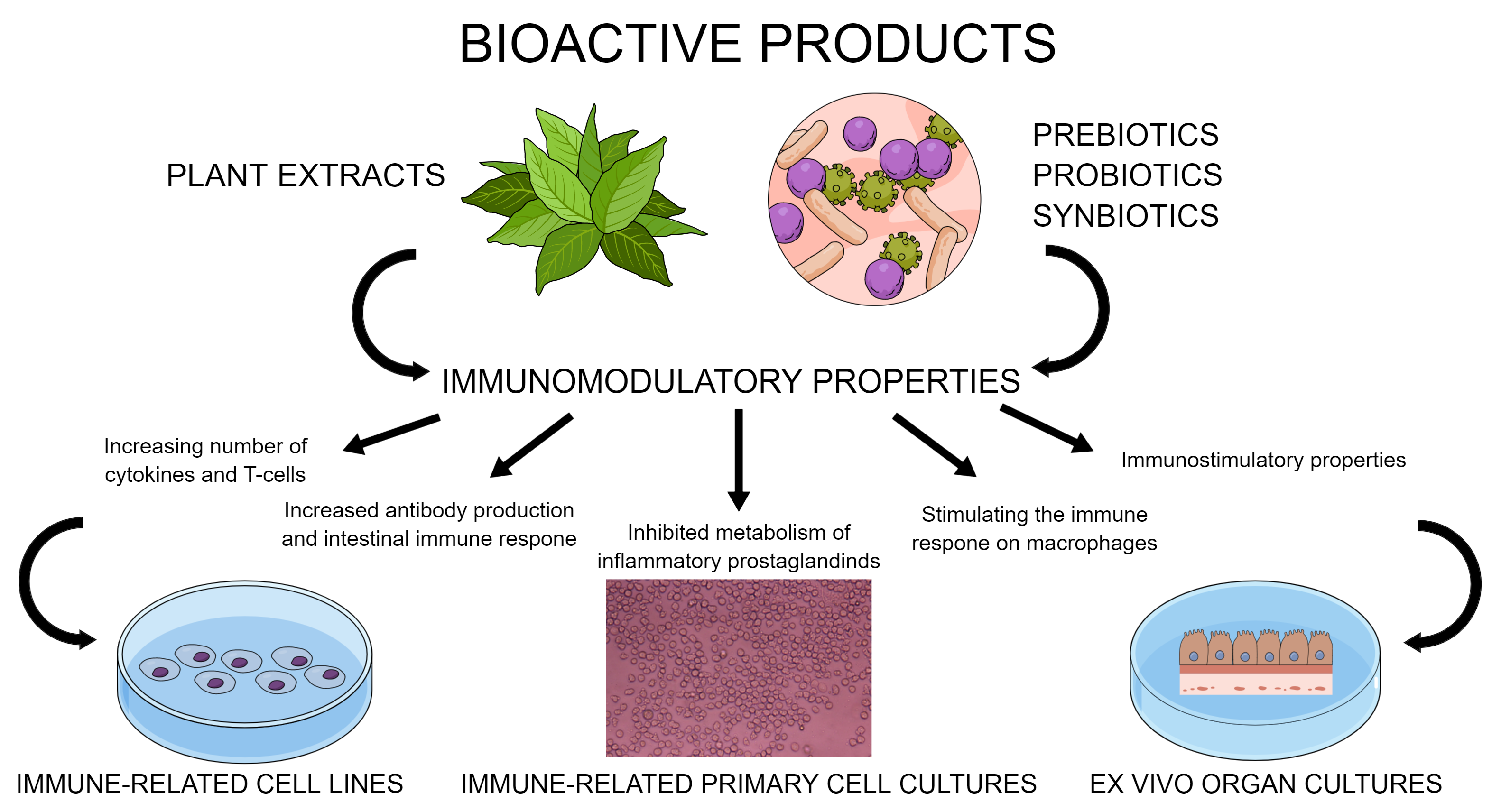The image is a detailed scientific illustration titled "Bioactive Products." At the top left, there is a depiction of a cluster of green leaves labeled "Plant Extracts." To the right of the plant extracts, enclosed in a circle, are icons representing "Prebiotics," "Probiotics," and "Symbiotics." Arrows connect these elements to the term "Immunomodulatory Properties." Further arrows from "Immunomodulatory Properties" highlight functions such as "Increasing Number of Cytokines and T-Cells," "Increased Antibody Production and Intestinal Immune Response," and "Inhibited Metabolism of Inflammatory Prostaglandins." To the right are arrows pointing to "Immunostimulatory Properties" and "Stimulating the Immune Response on Macrophages."

Below these, three additional depictions are shown. On the left, labeled "Immune-Related Cell Lines," is an image resembling petri dishes containing round, amoeba-like cells with cranberry-colored centers. In the middle is a pinkish rectangle with dotted patterns, labeled "Immune-Related Primary Cell Cultures," also resembling amoebas. On the right, within a petri dish, is a depiction labeled "Ex Vivo Organ Cultures," signifying a cultured organ environment. This comprehensive diagram showcases various bioactive products and their associated immunological impacts.